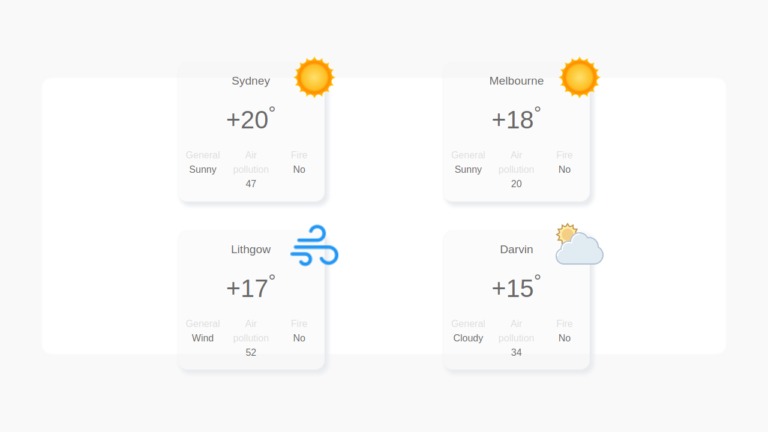This image is a horizontal screenshot with a faint, nearly indiscernible, light gray border. The background inside the border is white. Centrally located within the image are four square boxes displaying weather information for different cities.

The top left box is labeled "Sydney" and shows a temperature of +20 degrees. A bright yellow and orange sun icon is located at the top right corner of this box, indicating sunny conditions. Beneath the temperature, it says "General: Sunny." The air pollution level is listed as 47, and it states that there is no fire risk.

To the right, the next box is labeled "Melbourne," with a temperature of +18 degrees. It also features the same yellow and orange sun icon, signifying sunny weather. It reads "General: Sunny," with an air pollution level of 20 and no fire risk.

The bottom left box is labeled "Lithgow" and shows a temperature of +17 degrees. This box has a wind icon consisting of three blue lines that curl at the end, located at the top right corner. Below the temperature, it notes "General: Wind." The air pollution level here is 52, with no fire risk.

The final box on the lower right is labeled "Darwin," showing a temperature of +15 degrees. It features an icon of a cloud with the sun peeking out from behind it, indicating cloudy weather. It reads "General: Cloudy." The air pollution level is 34 and there is no fire risk.